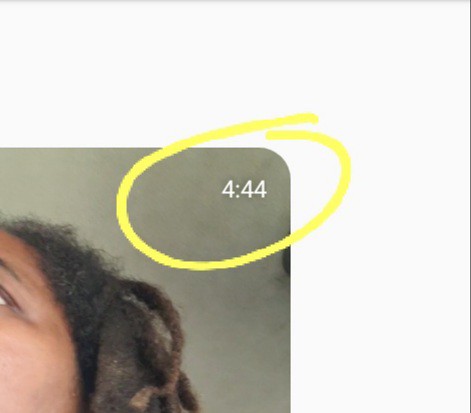The image depicts the partial photograph of a phone screen, specifically capturing the upper right corner which presents itself as slightly curved, consistent with a modern phone's display. At the top right of the screen, the time "4:44" is prominently displayed in white and encircled by a light yellow marker. The background is a muddled, greyish-green hue. Dominating the lower left corner of the photograph is part of a person's face, characterized by a dark complexion, with visible features including just the corner of their eyebrow and eye. They have distinctive afro-textured hair, notably with a long, matted strand tied off to the side. The photograph appears to have been taken at an angle where the person's face occupies the lower left to the central part of the phone screen diagonally, cutting through about a third from the left and extending halfway down.